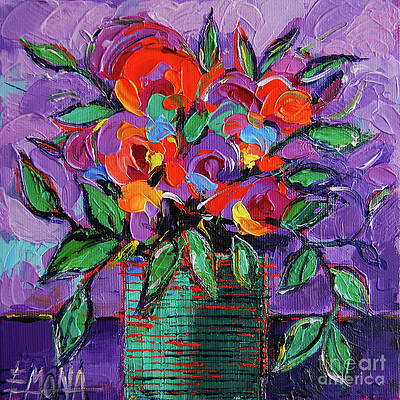This image is a close-up photograph of a richly textured painting depicting a vibrant floral arrangement in a green vase. The vase is broad and short, adorned with red and black stripes. Emerging from it are an array of flowers in shades of red, orange, purple, and hints of yellow, creating a vivid palette. The leaves vary in color, with those closer to the center being light green outlined in dark green, while those nearer the edges show gradients of darker green with light accents. The background is a dynamic mix of pink, cyan, and various shades of purple, including violet splotches, with areas of cyan particularly noticeable on the left side. The painting showcases visible brush strokes, adding to its textured feel. Additionally, the left side of the painting features a signature by the artist Mona, and the right side includes a gray silhouette line art of America, likely indicating copyright.